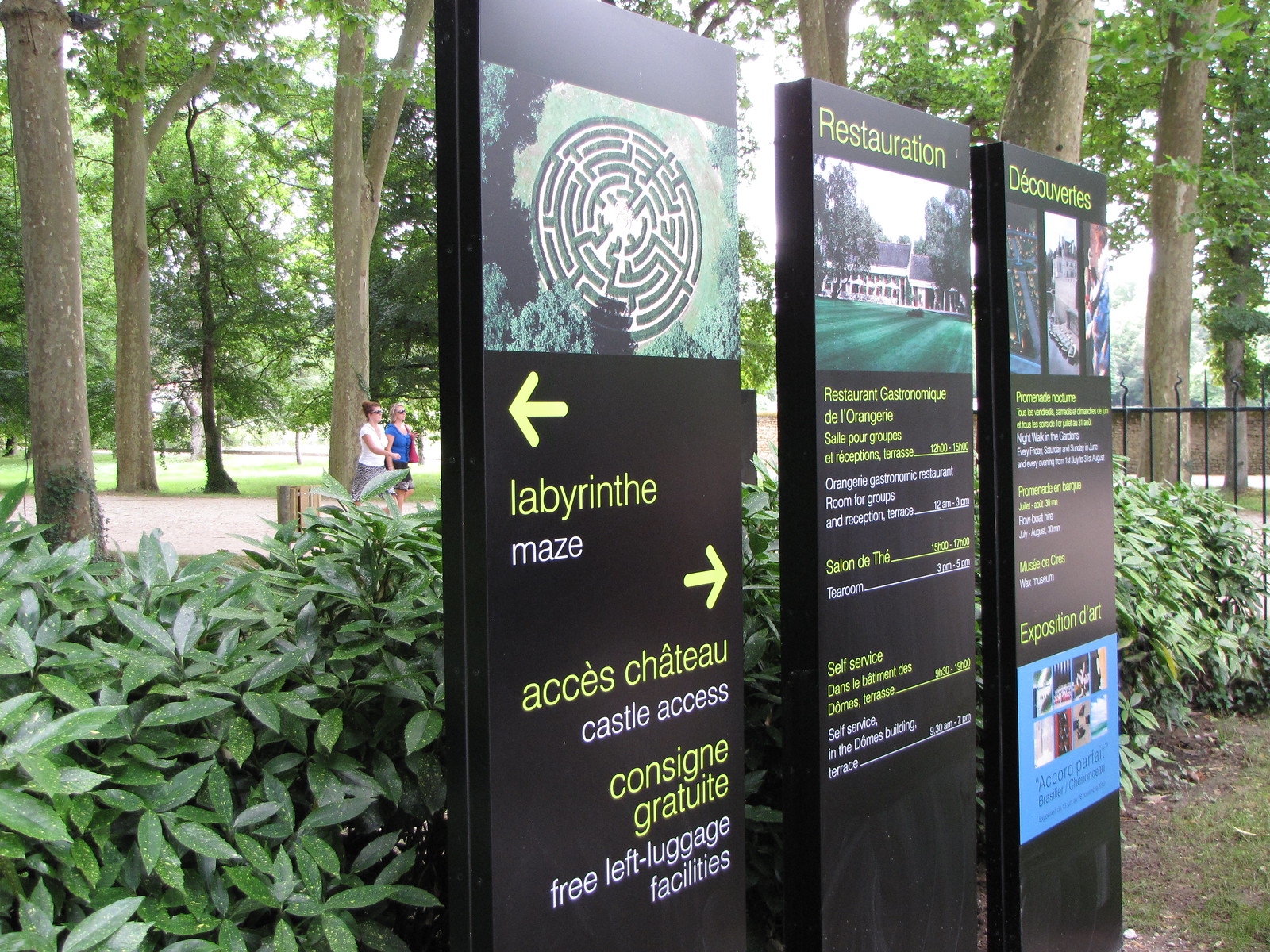The image captures three rectangular info banners in a forested area, featuring various attractions and facilities at what appears to be a restored castle tourist location. The signs are set against bushes with pathways, a trash can, and people walking in the background. The first sign directs visitors to a labyrinth maze, illustrated with a circular maze image, and provides directions to the castle and free left luggage facilities. The second sign lists dining options, including the Restaurant Gastronomique de l'Orangerie, with group rates, and specific times for the tea room and self-service dining in the Domes building. The third sign highlights additional attractions such as a night walk in the gardens available every Friday, Saturday, and Sunday in June, and nightly from July 1st to August 31st, a war museum, and a wax museum. There are also advertisements for a rowboat hire and an art show.